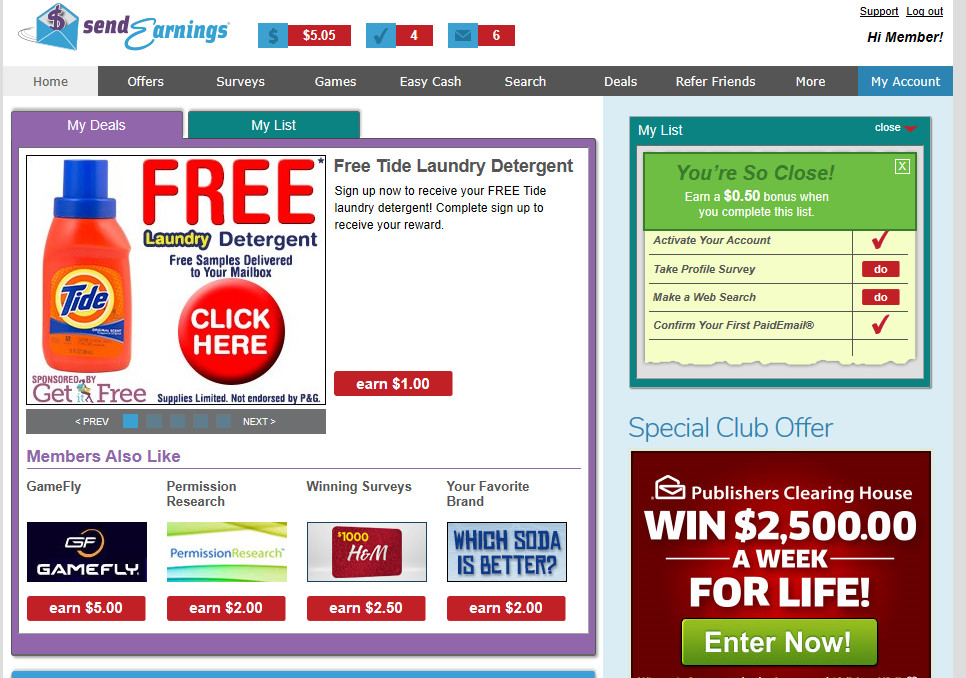The image depicts a digital interface resembling a local town newspaper filled with various coupon offers, somewhat similar to a "Sunday Saver." The screen is titled "Send Earnings" in the top left corner, suggesting it is part of an email chain or a website dedicated to money-saving opportunities. Central to the layout are several boxes displaying dollar amounts, checkboxes, and letter icons, likely indicating the number of coupons available and their values. 

The interface features multiple navigational tabs including "Home," "Offers," "Surveys," "Games," and "Easy Cash," bordering on resembling a platform designed for people to earn and save money through various activities. Prominently highlighted is a special offer for "Free Laundry Detergent," accompanied by a section labeled "Members Also Like" that lists additional monetizable offers. A notable "Publisher's Clearing House" advertisement is positioned in the bottom right corner.

The document also includes a list of daily tasks which presumably can be completed to earn bonus points. The overall design and content suggest that this might be an older interface, likely used by individuals aiming to save or make some extra money from home.